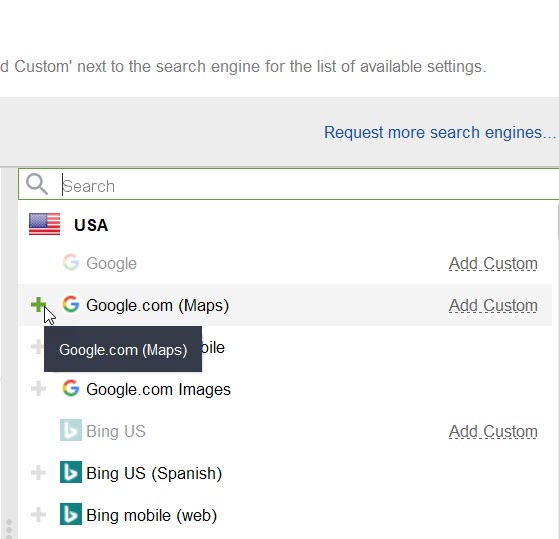The image depicts a user interface that appears to be a search engine management tool on a website. At the top of the interface, there is a gray box with the text "Request more search engines..." on the left-hand side. Beneath this box, there is a search field that indicates someone is conducting a personal search.

At the top of the main interface, there is a tab labeled "USA Search Engines." Under this tab, a list of search engines is displayed. The first entry listed is "Google," followed by "google.com," with the term "maps" in parentheses indicating a focus on Google's map services. The person’s cursor is hovering over a plus sign situated at the edge of this list. This plus sign is highlighted in green, implying that it is active or selectable, while the plus signs next to the other search engines remain gray.

Additionally, there is a black rectangle around the text "google.com/maps," emphasizing its selection. Below this entry are other search options: "US," followed by "US" in parentheses with the designation "Spanish," and another option labeled "Bing Mobile," with "web" in parentheses. This detailed depiction showcases the different search engine options available for configuration in the search tool.